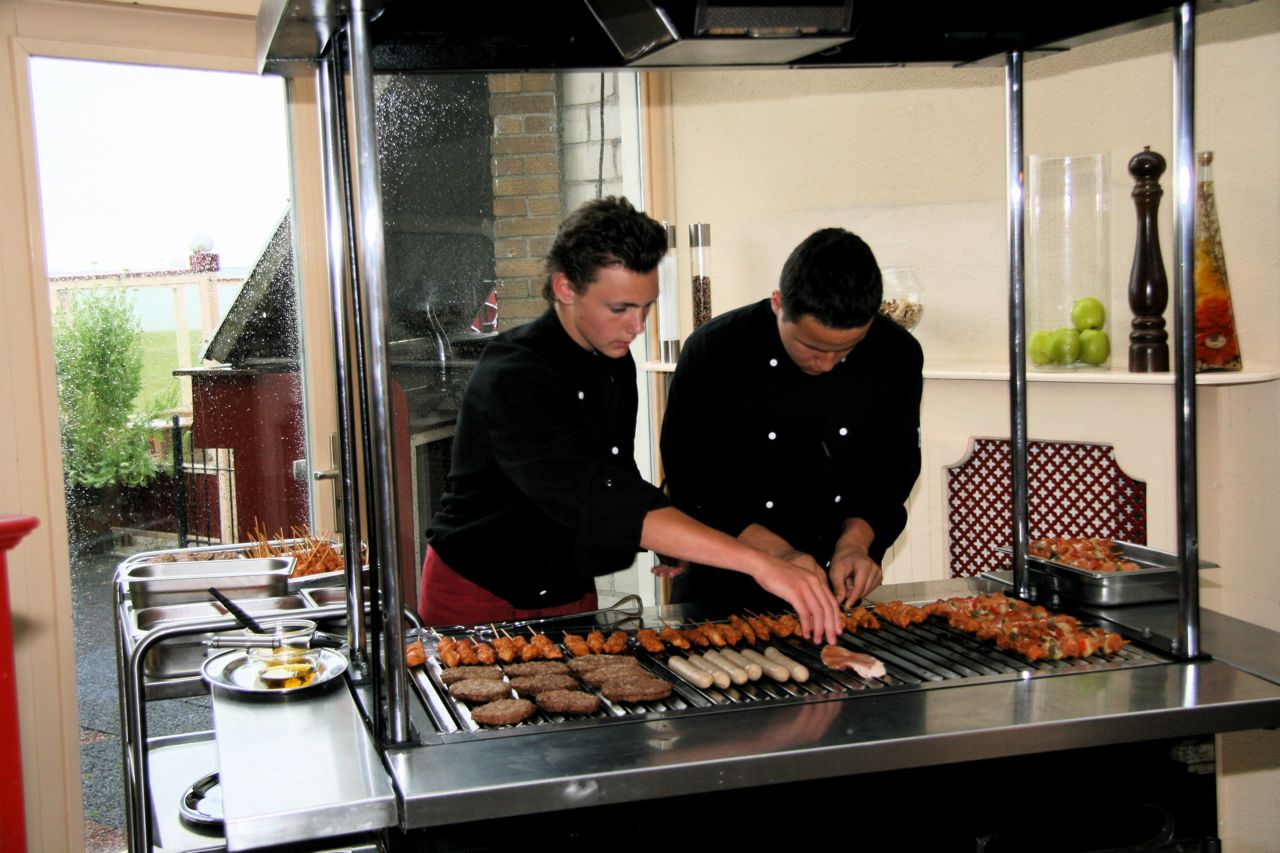In the photograph, two chefs wearing black vests with white double buttons, their sleeves rolled up, and red pants are intently working at a professional indoor grill setup. The chef on the right, with black, swept-back dark brown hair, bends over next to the chef on the left who has short, slightly curly black hair. Both chefs are diligently preparing an array of meats including sausage links, shish kebabs, and hamburgers on the large, silver rectangular grill, which is equipped with side tables for organizing their food. Behind them, additional trays of ingredients are prepared and ready for cooking. The professional kitchen setting is further accented by a large pepper mill and a jar possibly containing vinegar and oil dressing. Providing a glimpse of the outside, an open doorway on the right side of the image reveals trees against the sky.